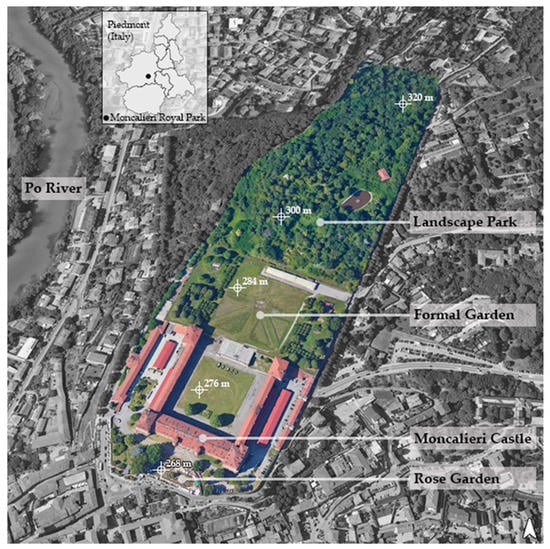This aerial photograph offers a detailed look at Moncalieri Royal Park, situated in Piedmont, Italy, as indicated by a legend in the top left corner. The park is bisected by the Po River, clearly labeled on the left side of the image. The park itself is prominently colored in vibrant greens while the surrounding cityscape fades into black and white, emphasizing the park's lush landscape. Key areas within the park are distinctly labeled: the expansive, wooded area of Landscape Park dominates the northern section, featuring dense clusters of trees and foliage. Directly below lies the meticulously manicured Formal Garden, comprised of refined lawns and neatly trimmed hedges. The imposing Moncalieri Castle stands at the southern end, characterized by its architectural complexity and red gabled roofs. Just in front of the castle, the Rose Garden adds to the botanical splendor of the park. Overall, the map illustrates a serene balance between natural woodlands and cultivated gardens, anchored by the historic castle at its heart.